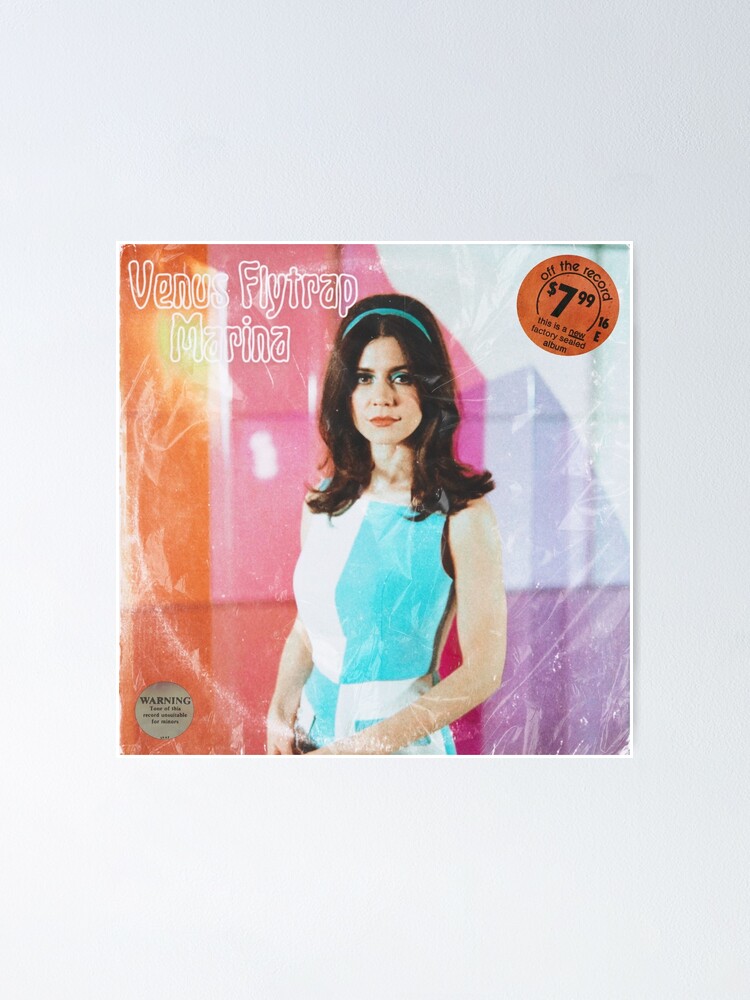This image depicts a factory-sealed vinyl record album cover resting on a grey background table. The album title, "Venus Flytrap Marina," is prominently displayed in the upper left corner in white, semi-transparent letters. Dominating the center of the cover is an image of a woman with long brown hair styled in a 60s fashion. She is dressed in a sleeveless blue-and-white dress, which matches her teal, aquamarine-colored headband and bright blue eyeshadow. The woman’s red lips and white skin stand out against a vibrant background swirled with pink, orange, and purple hues.

In the lower left corner of the album cover, there's a gold warning sticker with black text that reads, "Warning: Tone of this record unsuitable for minors." In the upper right corner, an orange sticker reads "Off the Record $7.99" with some smaller text below it. The cover also subtly reveals the imprint of the vinyl record inside.